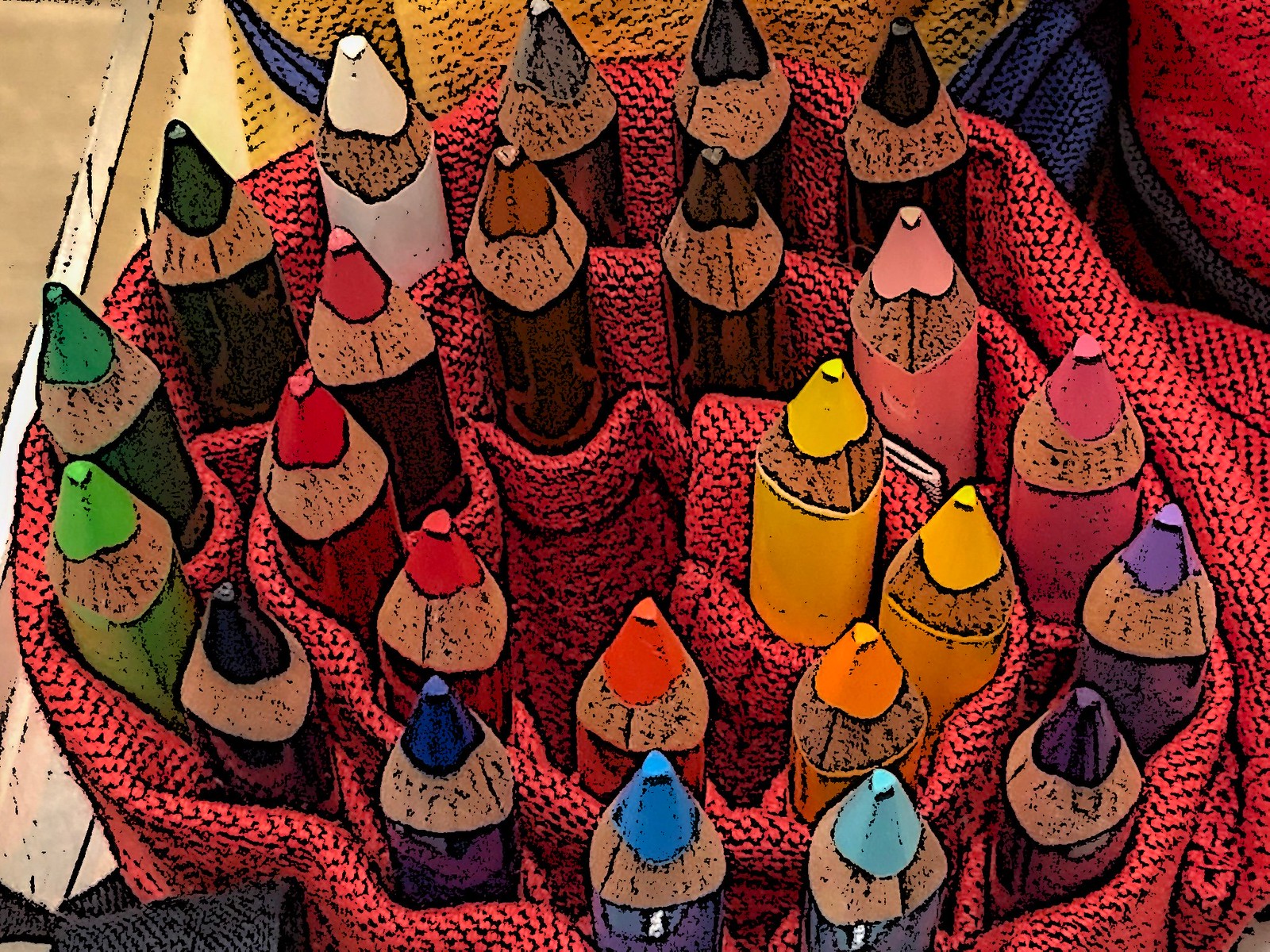The image appears to be a computer-generated illustration or a photograph with a filter, depicting a group of colored pencils organized in a spiral, rolled-up, pinkish-red cloth pencil holder. Each pencil is neatly placed in its own pocket, with their slightly dull but not heavily used tips facing upwards. The pencil holder, predominantly pink with hints of black weave, showcases a wide spectrum of colors ranging from black, through various shades of green, blue, purple, pink, brown, red, orange, to multiple hues of yellow. The pencils are not arranged in rainbow order but emit a vibrant, detailed, and visually appealing array of colors. The background suggests the holder might be placed in a wooden drawer, adding a rustic touch to the image.